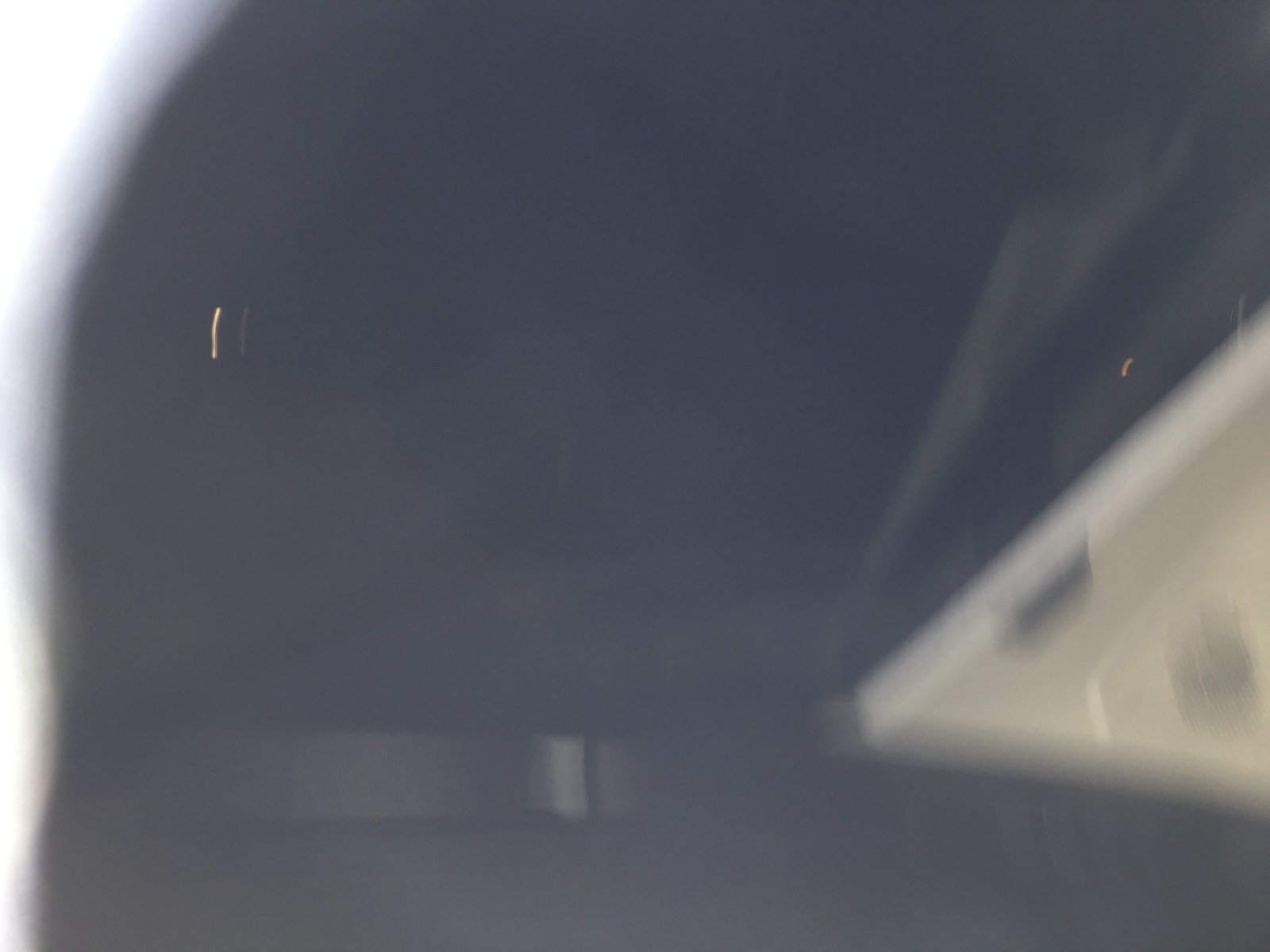A highly abstract, blurred photograph depicts a scene dominated by a dark, indeterminable surface that occupies most of the frame. This dark surface, which appears to have a tray-like shape, features elusive dark details crossed by what could be ribbons, belts, or lines, though the poor lighting obscures specific features. Below this dark expanse lies a white surface, lending contrast to the composition. To the left of the image, a bright light—possibly sunlight—illuminates the scene, casting reflections across the dark surface and creating ambiguous highlights. The overall atmosphere is shadowy, with the heavy blur and tight cropping preventing clear identification of the objects. The interplay of light and shadow lends a mysterious, almost ethereal quality to the image.